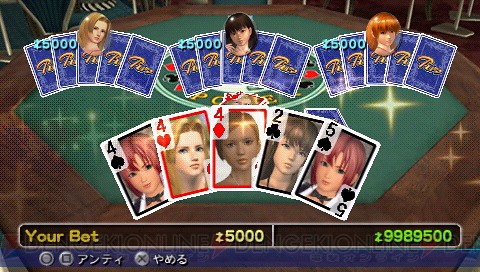The image appears to be a screenshot from a digital poker game, with game elements prominently displayed. The backdrop of the gaming screen is a brown, starburst-adorned surface, reminiscent of a casino table, partially covered with a green velvety section. Central to the game interface, the top third of the screen showcases three face-down, blue-backed card sets. Each set is marked with a bet amount of "5,000" and accompanied by distinct female avatars: a brunette, a black-haired girl, and a redhead, each enclosed in a circular or square frame.

In the lower portion of the screen, we see a player’s hand with five face-up cards, featuring charming cartoon-style female faces. The cards displayed are the four of spades, four of hearts, four of diamonds, two of clubs, and five of spades. Each card visually combines both suit and number with a character illustration.

Beneath the playing area, the bottom left corner of the screen states "Your Bet" in yellow, accompanied by the bet value "5,000." On the far right, another number "9,989,500" appears in a green box. Additional on-screen icons and Japanese lettering are present, enhancing the digital casino atmosphere of the game.